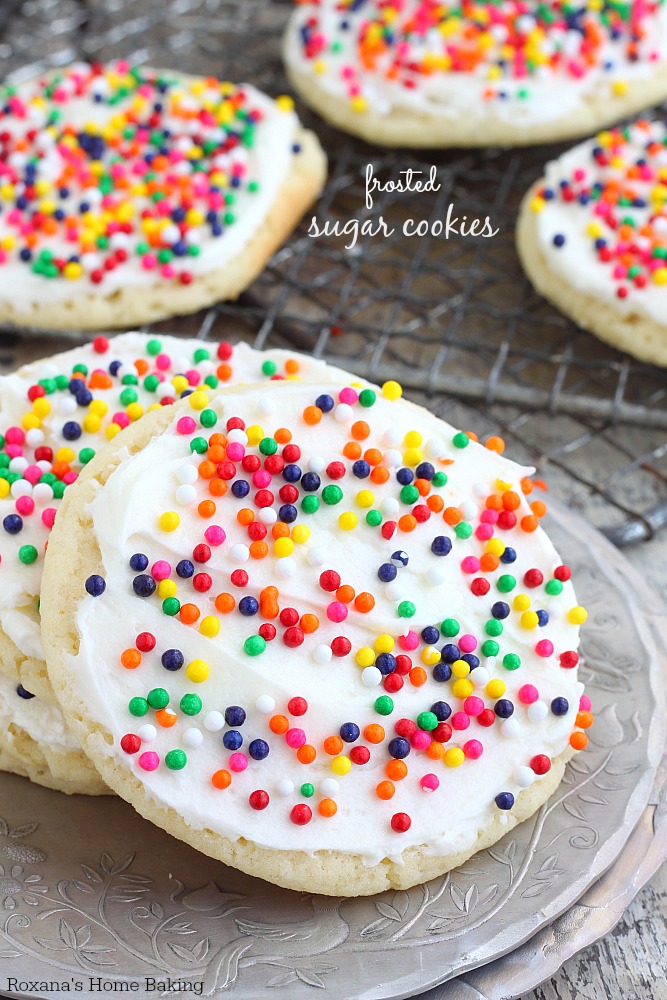In this color photograph, a collection of frosted sugar cookies is displayed, set against what appears to be a kitchen table. The cookies are light brown and round, lavishly coated with white frosting and adorned with multi-colored sprinkles in shades of red, pink, green, yellow, blue, black, and orange. The prominent text in the upper left corner reads "Frosted Sugar Cookies" in white script, while the bottom includes the words "Roxanna's Home Baking." In the foreground, we see two cookies, with one leaning against the other. They rest on what appears to be a silver or gray metal plate. In the background, there are three additional cookies partially visible, positioned on a silver baking rack that sits atop another mesh rack. The assorted colors and arrangements suggest a homemade or blog-like aesthetic, punctuated by the variety of vibrant hues throughout the image.